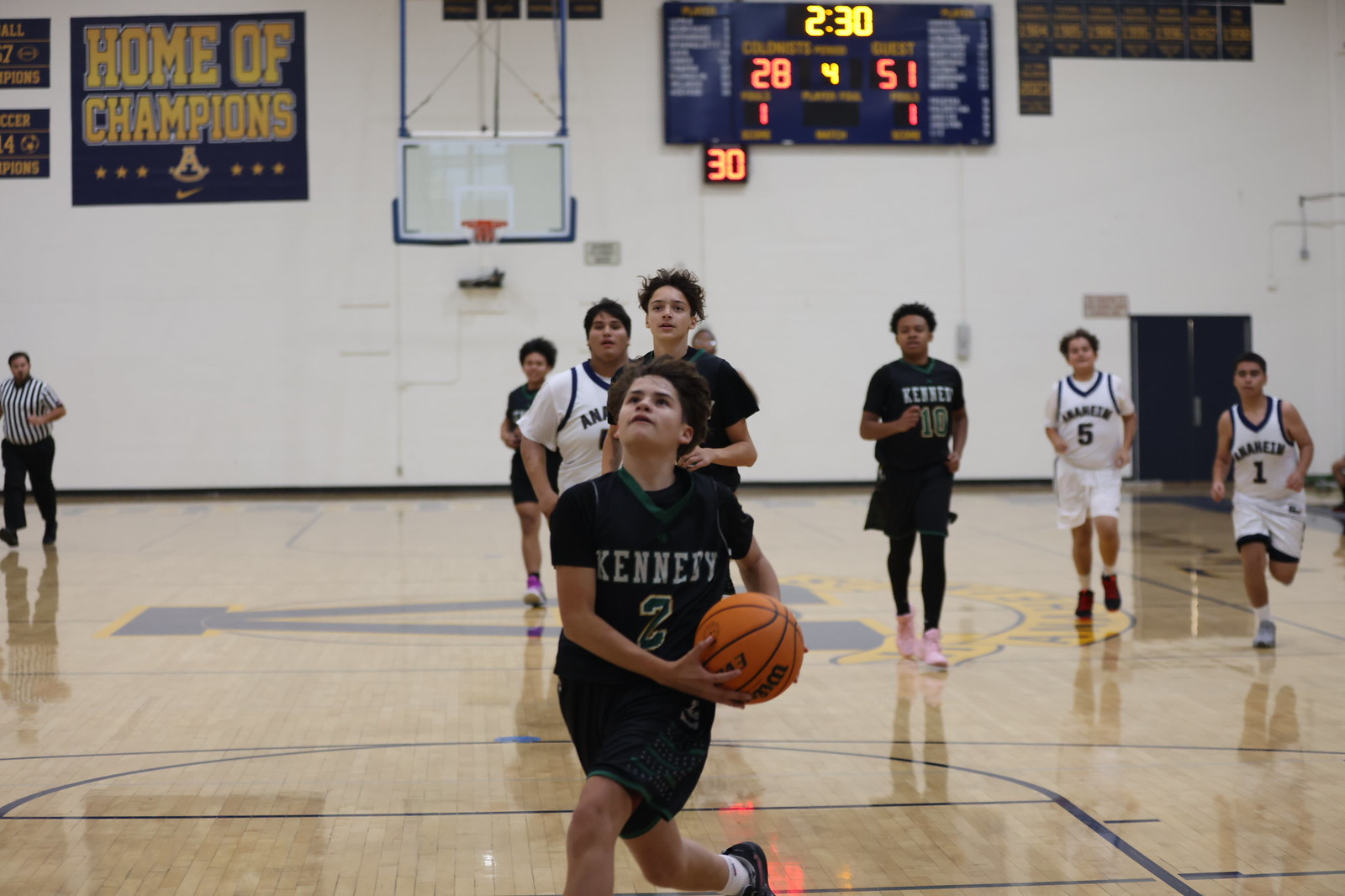The image captures a dynamic moment during a high school basketball game in a spacious gymnasium with polished wooden floors. Dominating the court is a large 'A' or 'V' logo at the center. The gym features white walls adorned with a prominent banner reading "Home of Champions" in yellow font against a dark blue-black background. A lit scoreboard displays the score 51-28 in the fourth quarter, with 2 minutes and 30 seconds remaining.

At the forefront, a youth player wearing a black jersey with green accents, white 'Kennedy' text, and a blue number '2' is captured mid-action, likely preparing for a layup. Eight players are visible on the court, divided into two teams: those in black jerseys with black shorts and the others in white jerseys with black accents. The referee, dressed in a striped black-and-white shirt and black pants, observes the action from the back left corner. The photo encapsulates the intensity and excitement of the game, with players and the referee fully engaged in the moment.